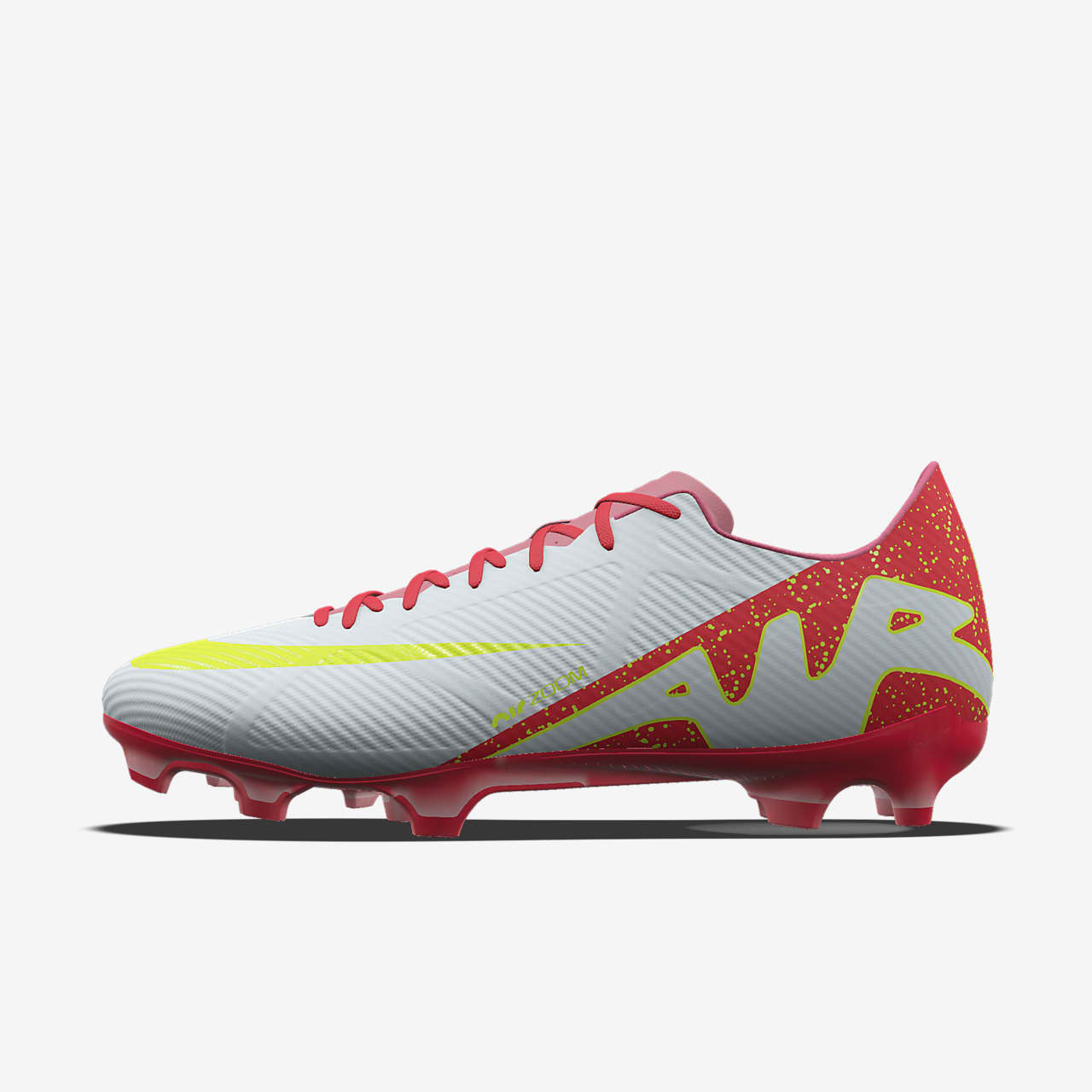The image showcases a white cleat positioned with the front end pointing towards the left and the back end towards the right, set against a white background. The cleat features a striking design with a white front, a red back adorned with yellow speckled dots, and an intricate yellow swirl pattern near the front. The back heel area prominently displays the word "AIR" in a fancy yellow-outlined white font. The sole of the shoe is red with plastic cleats. Red shoelaces and a matching red tongue accentuate the upper part of the shoe. Additionally, a yellow Nike swoosh is visible towards the toe, stretching diagonally across the side profile. The shoe is supported by an oval-shaped, dark gray shadow or frame beneath it, further grounding the image in a dramatic composition.